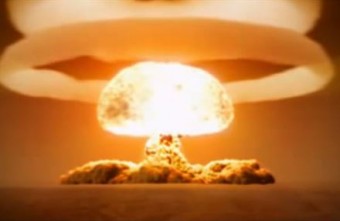The image depicts a small, square photograph, likely of an atomic bomb explosion, capturing a monumental moment of devastation. Dominating the horizon is a gigantic, bright mushroom cloud; its top part is an almost blinding white with hints of yellow and orange, emanating an intense, fiery glow. The explosion beneath the cloud presents a vivid display of red and orangish hues. The foreground, covered in reddish, rusty-brown dirt, meshes with a similarly colored sky, contributing to the overall surreal, monochromatic landscape. Above the prominent mushroom cloud hovers a massive, orangish smoke ring, seemingly suspended in mid-air. Additional lighter-colored smoke trails upwards, adding layers to this awe-inspiring, yet ominous scene. There is no text in the image, allowing the fiery, cataclysmic event to be the sole focus of this captivating photograph.